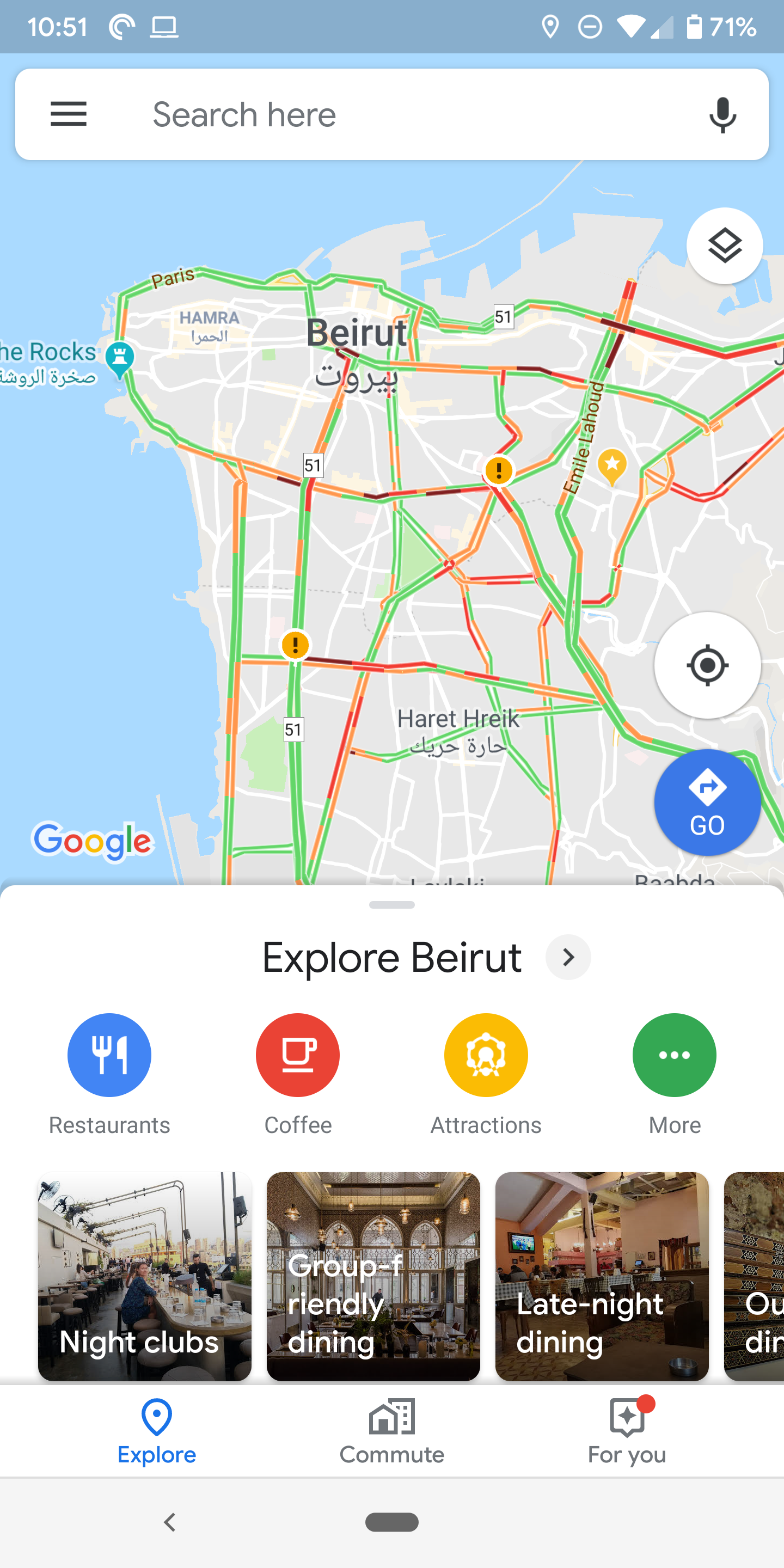This image is a detailed screenshot of a Google Maps search for Beirut. At the top of the screen, occupying the upper 5%, is the navigation bar displaying standard icons. The time is shown as 10:51, followed by an icon that resembles Comedy Central's logo ("CC"). Next to it, a laptop icon suggests the device is connected to a computer, and adjacent to that is the location pin icon. The "Do Not Disturb" icon is visible next, indicating the feature is activated. Following that, there are full Wi-Fi signal bars, a connectivity indicator showing 25% service strength, and a battery icon indicating 71% battery life.

Below the navigation bar is the search bar set against a white background, featuring the hamburger menu on the left, a search field labeled "Search here," and a microphone icon to the right for voice input.

The main portion of the screen displays a map of Beirut with roads color-coded to indicate traffic conditions—green for light traffic, yellow for moderate, and red for heavy congestion. In the bottom-left corner of the map image, the Google logo is present in its customary blue, red, yellow, and green colors. To the right of the logo is a blue navigation icon marked "Go." Above this is a target icon used for pinpointing the current location, and above that is the layers icon for adjusting map views.

At the bottom of the screen, a section titled "Explore Beirut" is present with icons representing categories such as restaurants, coffee shops, attractions, and more, each color-coded in blue, red, yellow, and green. Below these icons are image tabs that highlight options like nightclubs, group-friendly dining, late-night dining, and what appears to be hourly dining options. Further down are sections for "Explore," "Commute," and "For You," each accompanied by relevant icons. Finally, at the screen's very bottom is the home button for the phone interface.